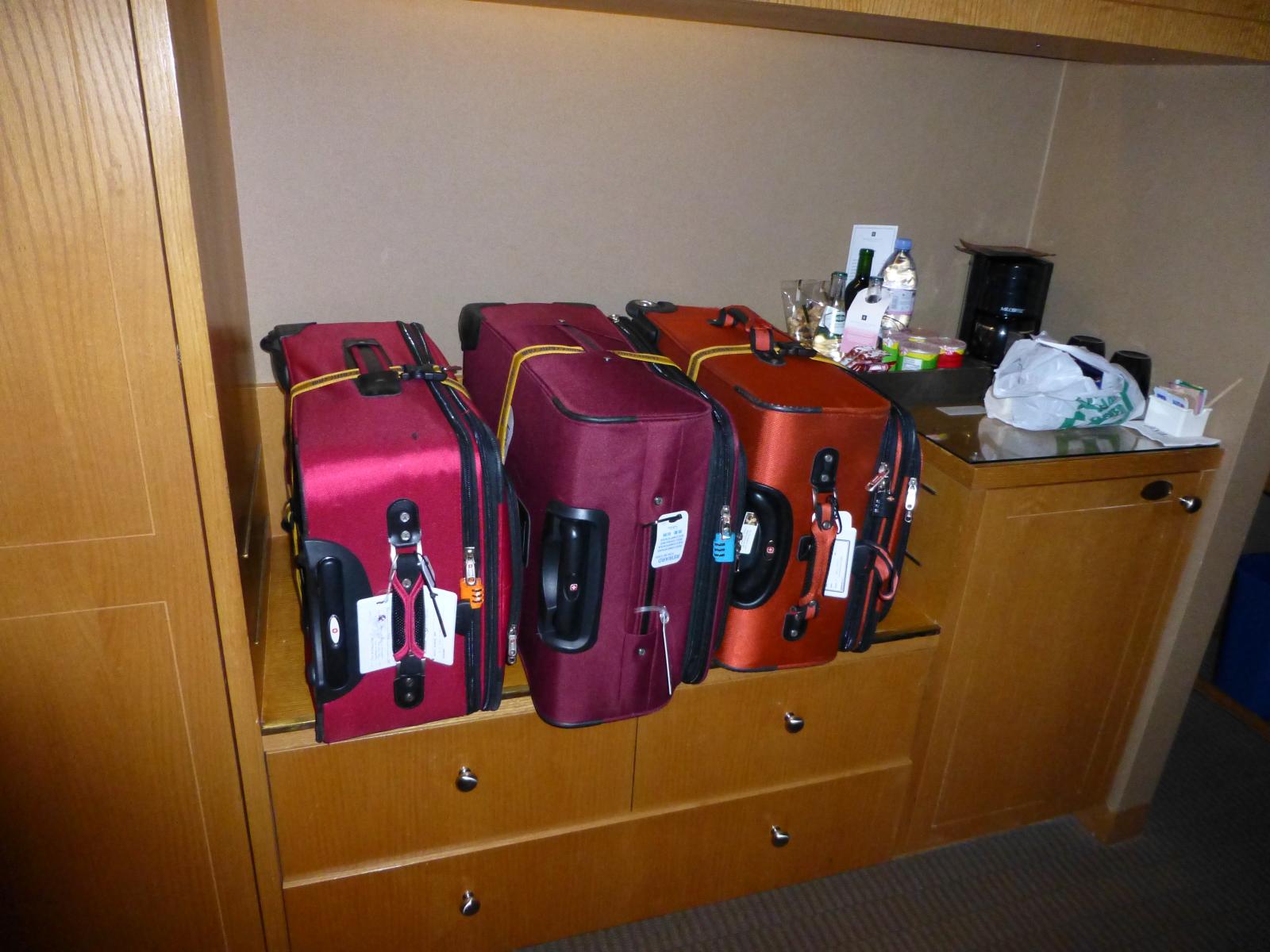This photograph, taken in a hotel room, displays a built-in dresser and a cabinet against a wooden backdrop. The dresser features a small, glass-topped counter in the corner, which supports a coffee machine and a tray containing water, cream, and sugar packets. Adjacent to this, there's a tall cabinet suitable for hanging clothes. Three nylon, roller-wheeled suitcases— one hot pink with a black border, one purplish maroon with a black border, and one hot orange—are neatly stacked side by side on the dresser. Each suitcase is secured with a bungee cord around the middle, suggesting they are still closed from travel. Below the counter, the dresser includes two small drawers and one large drawer for storage, while a white grocery sack is visible atop the counter. The overall layout and amenities, including two coffee cups, hint that this is indeed a hotel room catering to its guests' convenience.